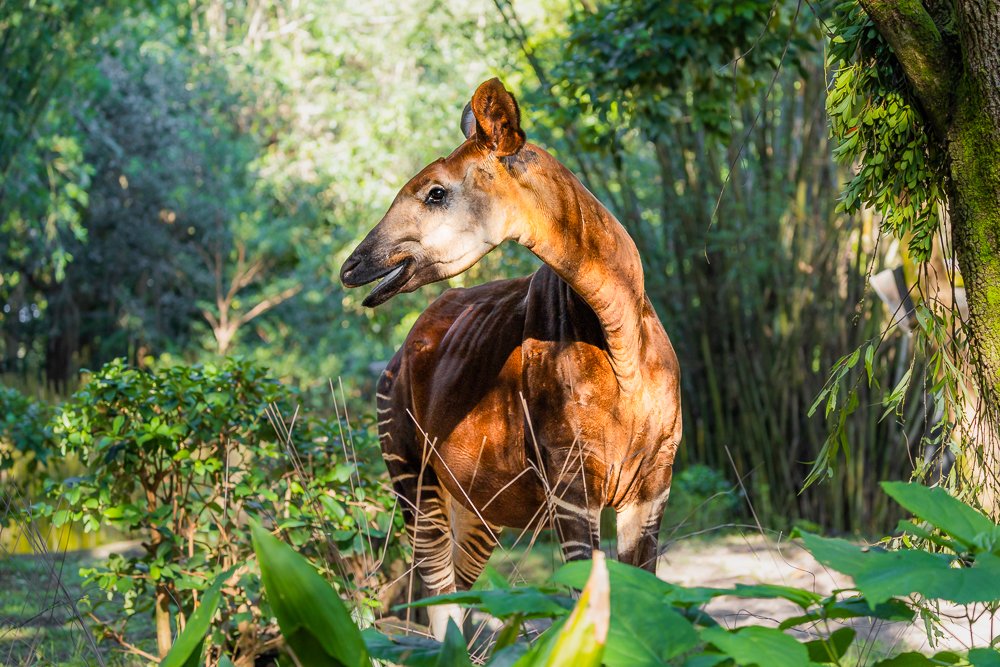In this image, we see an okapi, a unique animal that looks like a mix between a giraffe and a zebra, standing amidst a dense forest. The okapi's face, which resembles that of a giraffe but with a shorter neck, is prominently featured as it sways slightly to one side. The creature's distinctive patterning of stripes on its legs is partially visible. The background is rich with greenery, including bushes, small trees, and a variety of leaves, creating a natural, lush environment that highlights the okapi's presence.